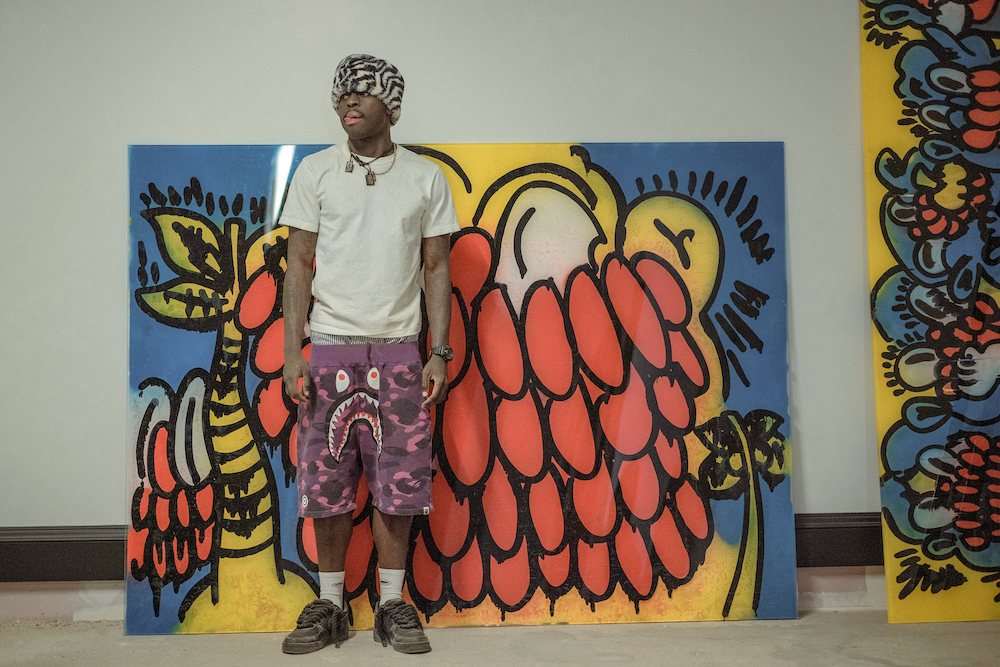In this vibrant photograph, a young African-American painter showcases his unique artistic flair. The man, sporting a playful expression with his tongue sticking out, wears a fuzzy black and white hat that almost covers his eyes. His casual outfit includes a white T-shirt, a pair of purple camouflage shorts adorned with a cartoon frowny face, and somewhat dirty black sneakers paired with white socks. His shorts hang low, revealing white and blue striped boxers underneath. Accessories include a couple of necklaces with medallions and a black watch on his right wrist.

He stands confidently in front of two large, vividly colorful paintings. The painting immediately behind him features a fantastical character reminiscent of a crazy clown or possibly Bart Simpson, with a mix of blue, pink, yellow, and white hues. Striking red shapes dangle off the character's face, adding a surreal, almost unsettling touch. To his right, a vertically-oriented painting with a yellow background depicts blue cartoon-like figures, possibly resembling monkeys with red markings on their faces and expressive eyes. This composition beautifully merges elements of pop art and street art, hinting at the painter's dynamic and rather eclectic creative vision.